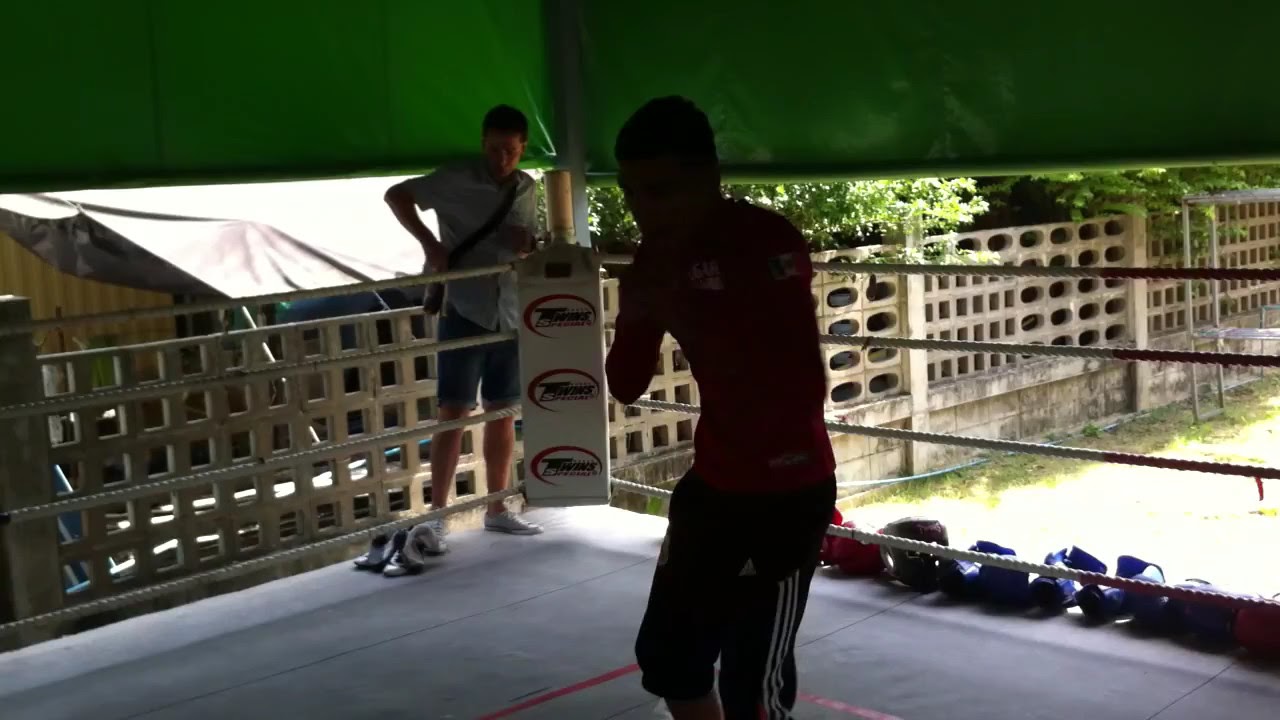In this vivid outdoor scene, we find ourselves inside a boxing ring set against a backdrop of stone fencing and lush green trees, sheltered by a partly lifted green canopy filtering in diffused daylight. The ring floor is gray adorned with red tape markings, bordered by white ropes and turnbuckles with unreadable text encircled in red. 

Prominently in the ring's corner stands a fighter wearing black Adidas pants with the iconic three white stripes on his left leg, paired with a red shirt that appears dark due to the lighting. Outside the ring, another man dressed in a white or gray button-down shirt, blue denim shorts, and white shoes holds a black-strapped bag over his shoulder, seemingly engrossed in something below - perhaps a phone. 

The ring's edge is lined with an assortment of gear, including blue and white gloves, black helmets, and red gloves, ready for sparring. Beyond the ring, a blue canopy and a silver painter's stand can be seen, contributing to the eclectic yet organized training environment. This detailed snapshot offers a glimpse into the organized chaos of a boxing training session taking place in a tranquil, shady outdoor setting.